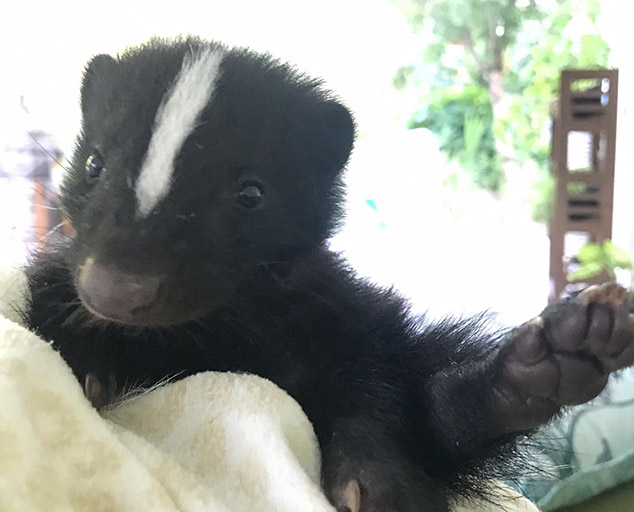This close-up outdoor color photograph captures an adorable baby skunk, wrapped snugly in a tan and white patterned blanket, as it's cradled in someone's arms. The tiny skunk, predominantly black with a distinctive white stripe running from its nose up through the center of its head, is gazing directly into the camera, with its head slightly tilted to the left and its black, beady eyes wide open. Notably, the skunk's left paw is extended, revealing detailed features of its foot at the right side of the image. The background is mostly washed out and white, suggesting a very sunny day, with faint hints of greenery and possibly a tree or shelving unit in the backdrop, contributing to the outdoor setting. The intimate framing and clarity of the image emphasize the skunk's delicate features and the tender moment of being held, highlighting its youthful and clean appearance.